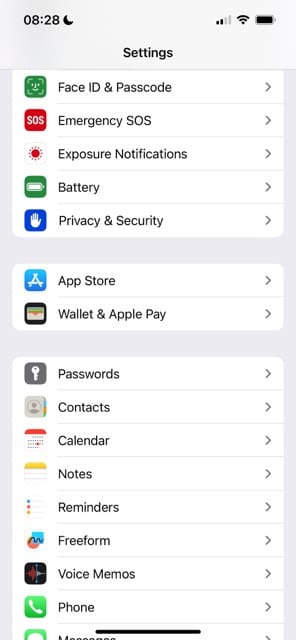### Detailed Caption for Settings Screenshot:

This is a screenshot of the settings menu on a phone, capturing the following details:

- **Top Bar:**
  - The time displayed is **8:28**, written in black text.
  - To the right of the time is a black icon of a moon, indicating that the device is likely in **Do Not Disturb** mode.
  - Icons for **Wi-Fi signal strength** and **full battery** are also visible.

- **Header:**
  - The word **"Settings"** is prominently written in black at the top of the screen.

- **List of Settings Options:**
  - The first option is labeled **"Face ID & Passcode"**. It is accompanied by a small green box with white writing that forms the shape of a face.
  - The next option is **"Emergency SOS"**. It features a red box with white writing saying "SOS".
  - Following that is **"Exposure Notifications"**, indicated by a white box with a red sun icon.
  - The setting for **"Battery"** is noted with a green box containing a white battery icon next to black text.
  - The section labeled **"Privacy & Security"** includes a blue box with a white hand icon.
  - The **"App Store"** option is identified with the App Store icon next to it.
  - Additional settings are listed below, in black text:
    - **Wallet & Apple Pay**
    - **Passwords**
    - **Contacts**
    - **Calendar**
    - **Notes**
    - **Reminders**
    - **Freeform**
    - **Voice Memos**
    - **Phone**, marked with a green square containing a white phone icon.

This organized screenshot presents a clear overview of various critical settings available on the device, using a combination of text and iconography to distinguish each category.